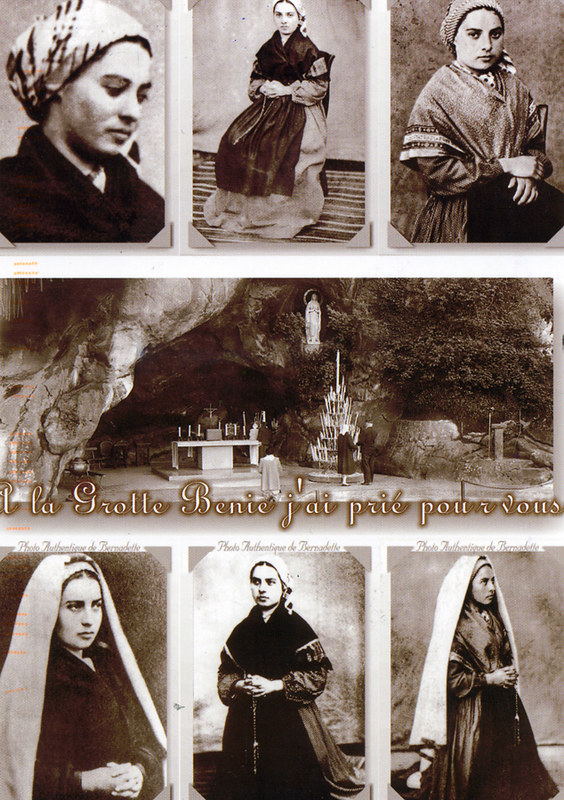This image is a collage of vintage, black-and-white photos formatted into a portrait-oriented rectangle. At the top, three photographs of a woman in ethnic costume display her in a close-up wearing a scarf or hood, sitting on a chair draped with a long scarf, and looking straight ahead. Each photo is framed in the corners. The middle section features a horizontal image of a grotto or cave with rock formations, kiosks, religious statues in niches, and people milling about. French or another foreign language text, partially cut off, reads "La Rue, Venice, Paris, Porto." The bottom row presents three more photographs of the same woman in different poses, all wearing traditional head coverings, shawls, and long skirts. These photos, slightly sepia-tinted, reinforce the vintage aesthetic, combining early photography with graphic design elements.